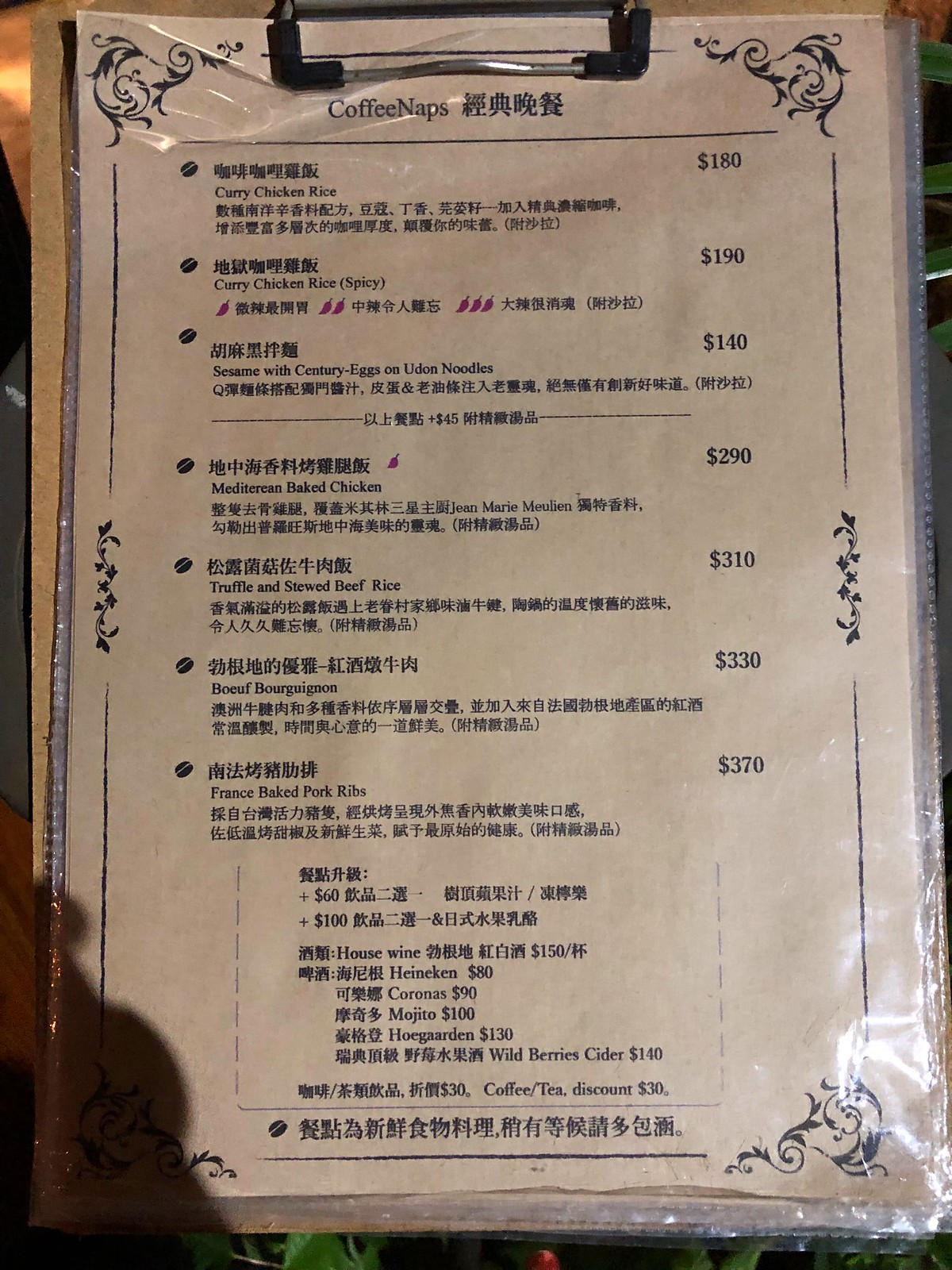The image showcases a restaurant menu titled "Coffee Naps," written as a single word. The menu features both Asian characters and English text, though the specific language of the characters is not indicated. Below these characters, there are detailed listings of menu items in English, including "Curry Chicken Rice," "Sesame with Century Eggs," "Mediterranean Baked Chicken," and "Truffle and Stewed Beef Rice."

Notably, the prices listed seem extraordinarily high, with "Curry Chicken Rice" priced at $180, a Heineken beer at $80, and a Hoegaarden beer at $130. Given the presence of a dollar sign next to these amounts, it suggests either this is a very high-end establishment or the menu prices are listed in a local currency that uses the dollar symbol, which might differ from common understandings of pricing.

The overall impression is a distinctive blend of Asian and Western culinary offerings in a setting where the local currency might explain the seemingly inflated prices.